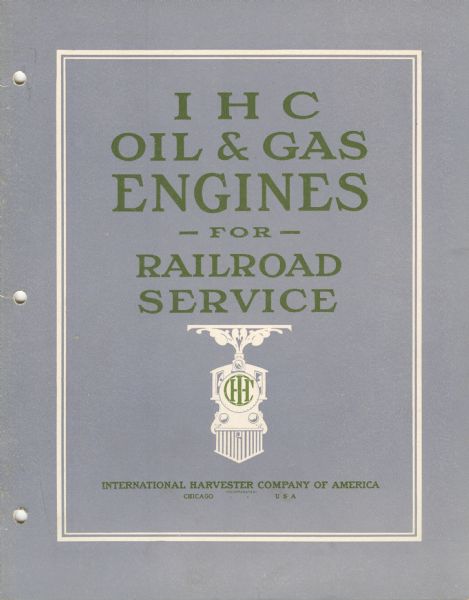This detailed image features an old instruction manual or binder cover predominantly blue in color, designed for IHC oil and gas engines used in railroad service. The manual, which is likely from a three-ring binder as indicated by the three holes punched on the left-hand side, presents a distinct layout. 

At the top, bold green letters spell out "IHC oil and gas engines for railroad service" against a white background. Below this title is a prominent illustration of a white locomotive facing directly forward, steam visibly emitting from its exhaust pipe. The locomotive's front grille features the initials "IHC" amid a pattern of green lines contrasted against a yellow background. 

Adding to the informative nature, the bottom of the cover highlights the text "International Harvester Company of America, Chicago, USA," signifying its American origin. The cover is further framed by a white interior border and a tan border, providing a structured and classic appearance indicative of historical industrial literature.